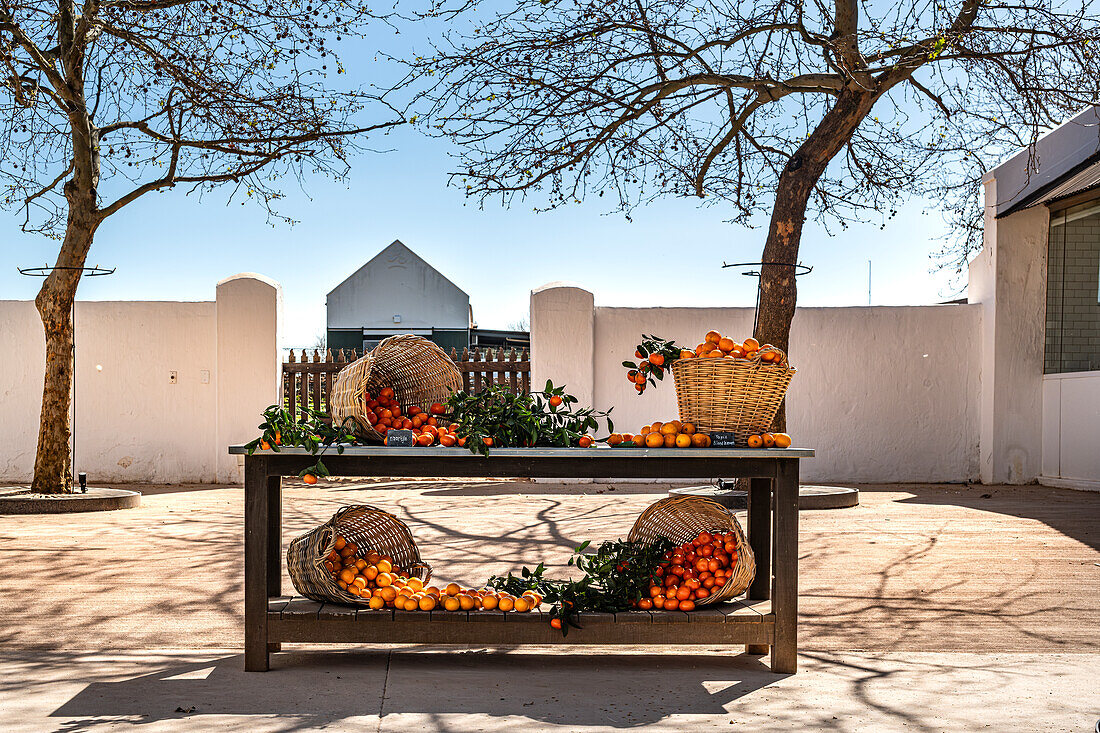The high-resolution photograph captures a detailed scene of a table made of dark gray wood situated outdoors in a courtyard under a clear blue sky. This table, arranged in a two-tiered shelf style, supports a vivid display of oranges across four baskets. On the top level, one basket is upright and filled to the brim with vibrant oranges, while another basket is halfway tipped over, causing some oranges to spill onto the table. On the lower level, two more baskets are turned on their sides, sending yet more oranges cascading out. The total number of oranges appears to be at least 40, with some showing a yellowish-orange shade, contrasting against the predominantly bright oranges. Additional loose oranges and green, leafy objects are scattered on the table's surface, enhancing the sense of abundance. Behind the table, the courtyard features two tall, bare trees alongside a tall concrete fence and a brown wooden fence, which partially obscures a building with a sloped roof. The entire scene is bathed in natural daylight.